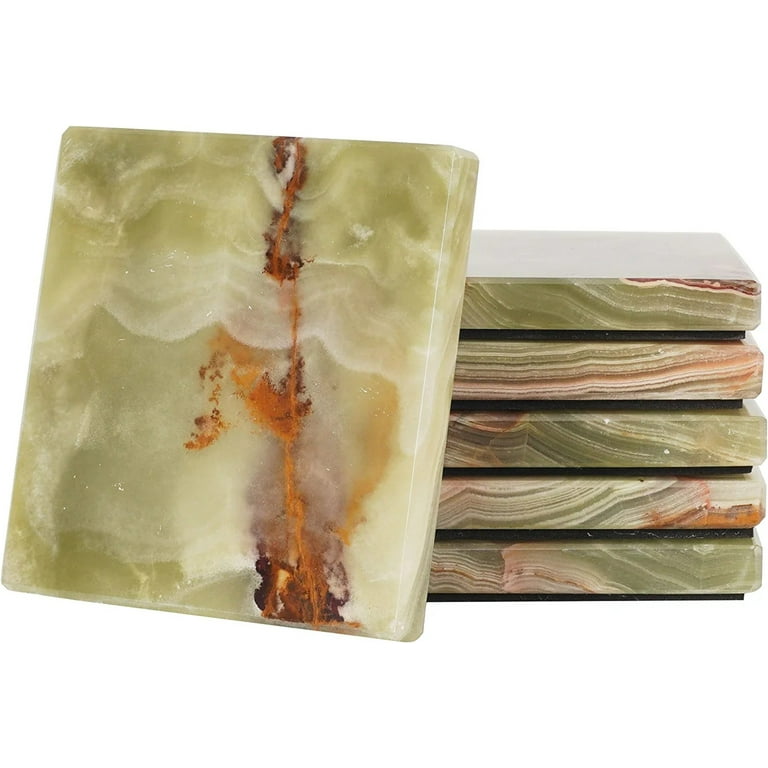The image showcases a set of six square marble coasters. Five of the coasters are stacked in a tower-like fashion on the right, while the sixth coaster is propped upright and leaning against the stack. Each coaster features a marbled design with a mix of colors, including light green, white, dark orange, brown, and hints of pink. The propped-up coaster prominently displays a brown, upside-down "J" shape near the top, bordered by dark green with white wavy lines reminiscent of ocean waves washing onto a beach. It also features a dark brown and darker orange patch at the bottom. The sides of the stacked coasters reveal a layered effect with the same color palette. The bottom appears to have a black grip material to prevent sliding or scratching surfaces, emphasizing their functional design as coasters.